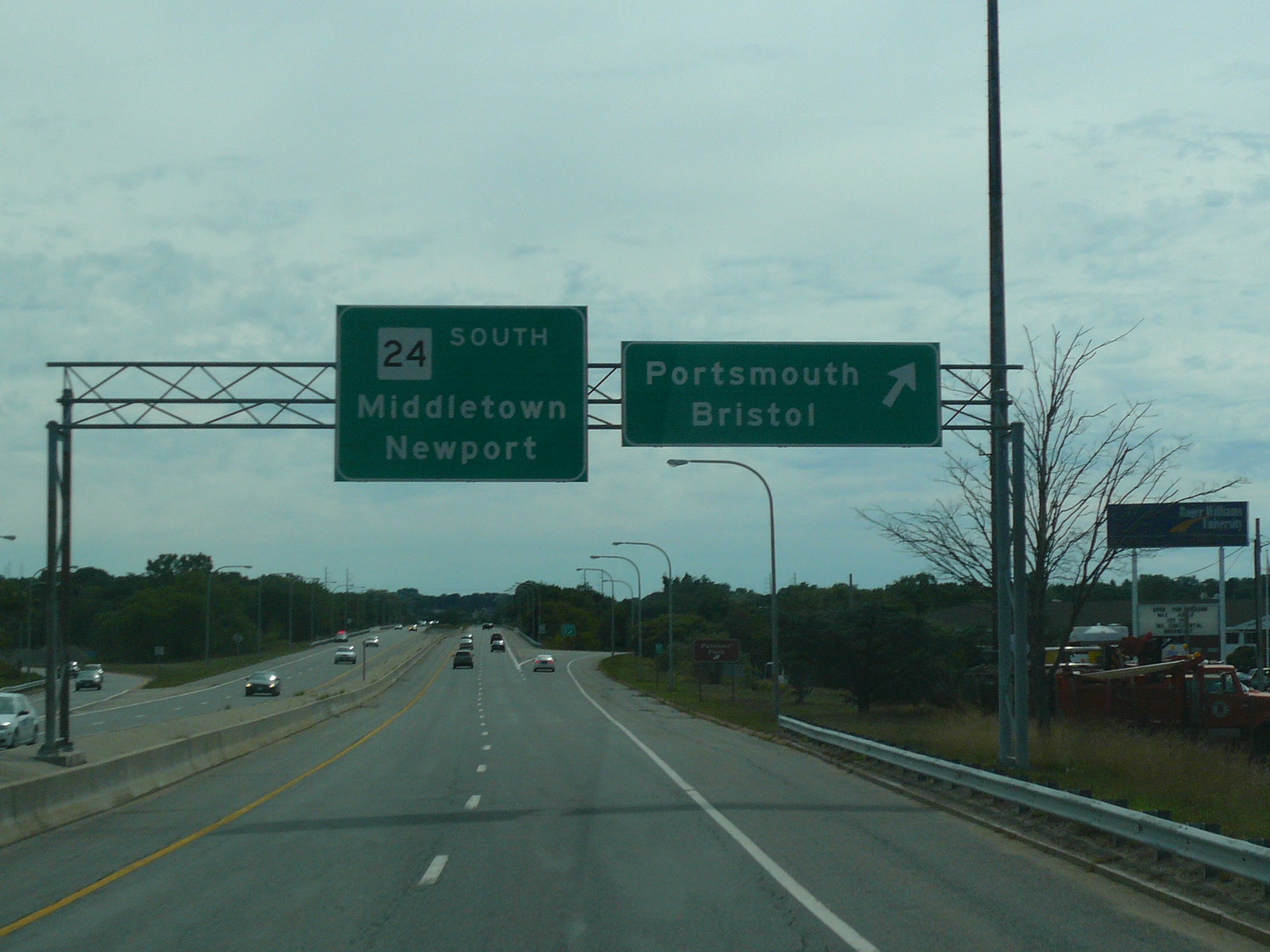This photograph depicts a relatively calm and uncrowded Highway 24. It features two lanes in each direction, delineated by dotted white lines in the center, a solid white line on the right, and a solid yellow line on the left. On the left side, an on-ramp merges into the highway, while to the right, a grass shoulder separates the road from a few stationary dump trucks. Spanning across the highway is a prominent pole with two green signs: the left sign contains the numbers "24" in a white box and the text "South Middletown Newport," while the right sign reads "Portsmouth Bristol" with an arrow pointing forward to the right. The day is notably overcast, contributing to a tranquil ambiance that hints at an ideal setting for a relaxed road trip, free from traffic congestion. In the background, there are two billboards; one advertises Roger Williams University, though the specifics of the other remain indistinct due to the image resolution.